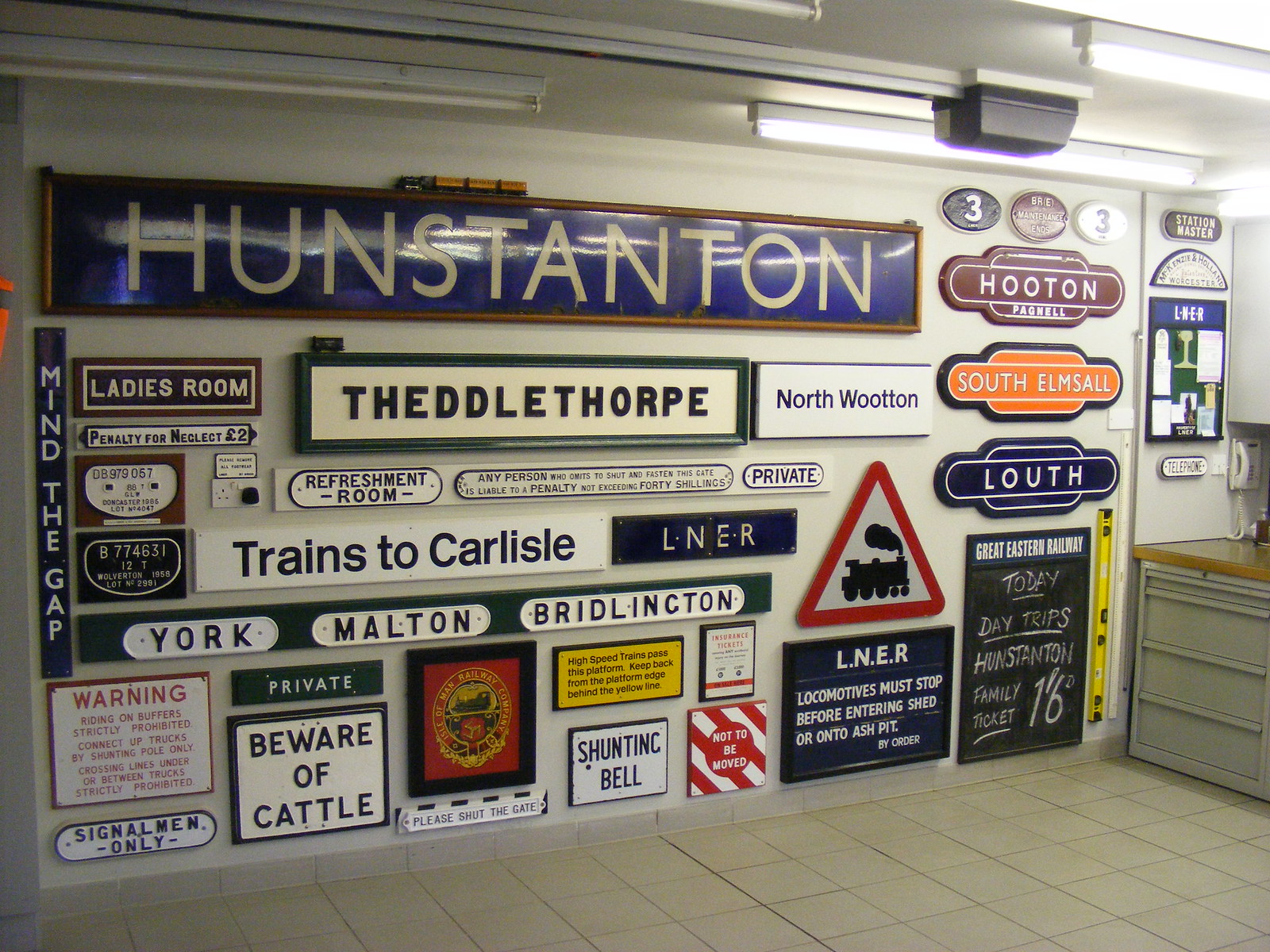The image shows an indoor scene, likely a museum exhibit, featuring a white tiled floor and a portion of a table or workbench on the right. Mounted on the wall is a corded phone with a sign labeled 'telephone' and a bulletin board above it. The walls are adorned with an array of vintage railway and informational signs. The most prominent sign is a long, blue rectangular one at the top with 'Hunstanton' in white print. Below it are several rectangular signs including 'North Wooten', 'Fetlethorpe', 'trains to Carlisle', 'ladies room', and 'beware of cattle.' Additional square signs at the bottom display messages such as 'signalman only' and 'shunting bell.' Other notable signs include warnings and directional indications like 'penalty for neglect two pounds', 'keep back from the platform edge behind the yellow lines', and 'LNER locomotives must stop before entering shed or on to ash pit by order.' These signs suggest the setting of a historical train station exhibit, emphasizing the careful curation of railway memorabilia.